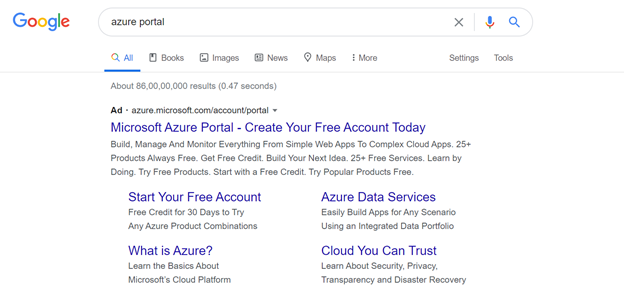This image is a screenshot of a Google search query for "Azure portal." At the top left corner, the Google logo is displayed with its characteristic colors: the big 'G' and small 'g' are in blue, the first 'O' and the 'e' are in red, the middle 'O' is yellow, and the 'l' is green with the second 'l' in blue.

Directly below the logo, a search bar contains the phrase "Azure portal." Under the search bar, a navigation menu features headings such as "All," "Books," "Images," "News," "Maps," "More," "Settings," and "Tools." The "All" tab is highlighted in blue and underlined, indicating the active selection, while the others remain in gray.

The search results display a single entry, labeled as an advertisement from Azure.Microsoft.com. This ad headline reads "Microsoft Azure portal - Create Your Free Account Today." The detailed ad text outlines the capabilities of the Azure portal, mentioning that users can build, manage, and monitor everything from simple websites to complex cloud applications. It highlights the availability of 25+ free products, the opportunity to get free credit, and the promotion to build your next idea using the free services.

The advertisement further encourages starting a free account with a 30-day credit to try various Azure products. It briefly answers "What is Azure?" by explaining it as Microsoft's cloud platform suitable for building apps for any scenario using an integrated data portfolio. The ad includes a final note on the reliability of Azure, emphasizing its security, privacy, transparency, and disaster recovery features.